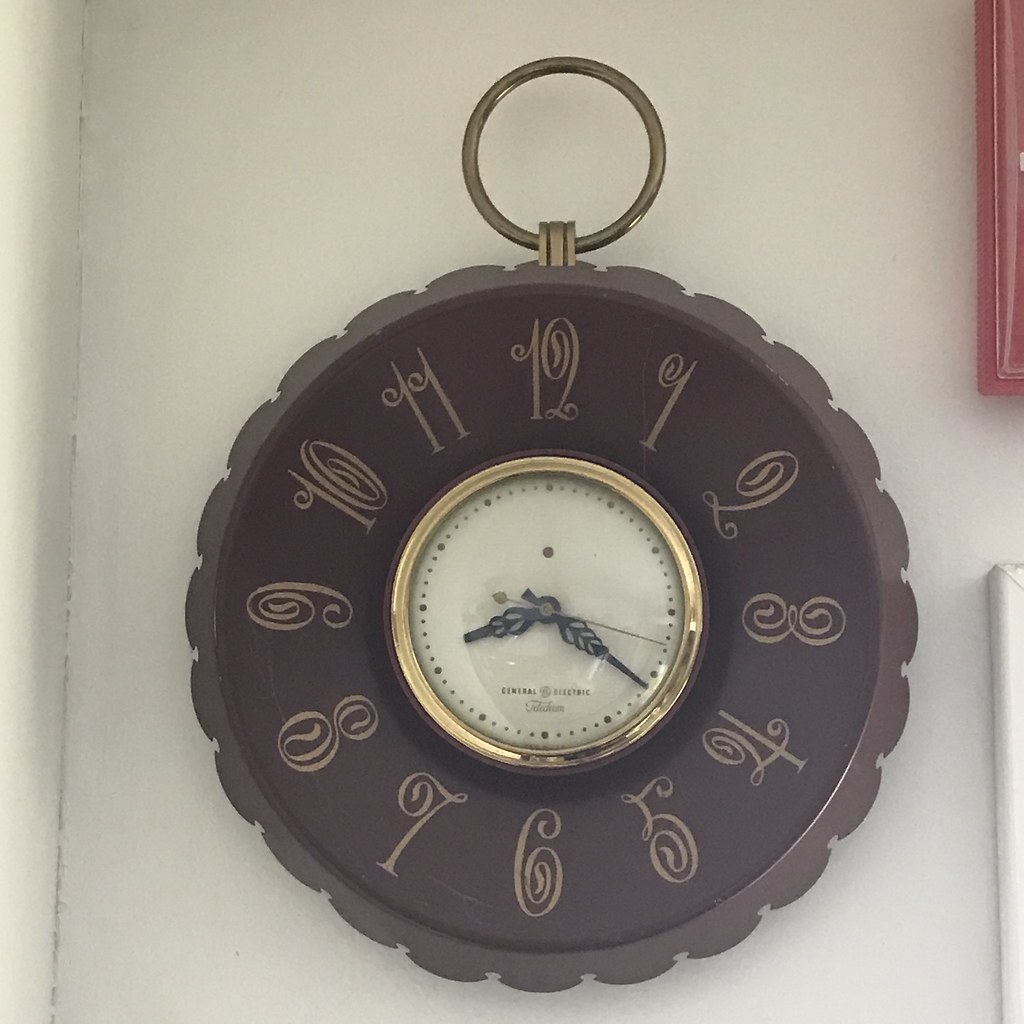The photograph features an antique wall-mounted analog clock with a predominantly dark maroon or brown hue. The clock face is white, encircled by a gold or brass edge, and it bears black minute and hour hands alongside a brass second hand. The clock displays the "General Electric" brand, likely with additional cursive writing too small to decipher. Surrounding this central face, the maroon portion includes large, ornate numbers from 1 to 12, painted in a fancy script style. At the top of the clock is a gold brass ring, resembling a keychain. The clock is set against a white wall, with a red and white picture positioned to its right. The overall aesthetic of the clock combines elements of brown and gold, reminiscent of a vintage or antique style.